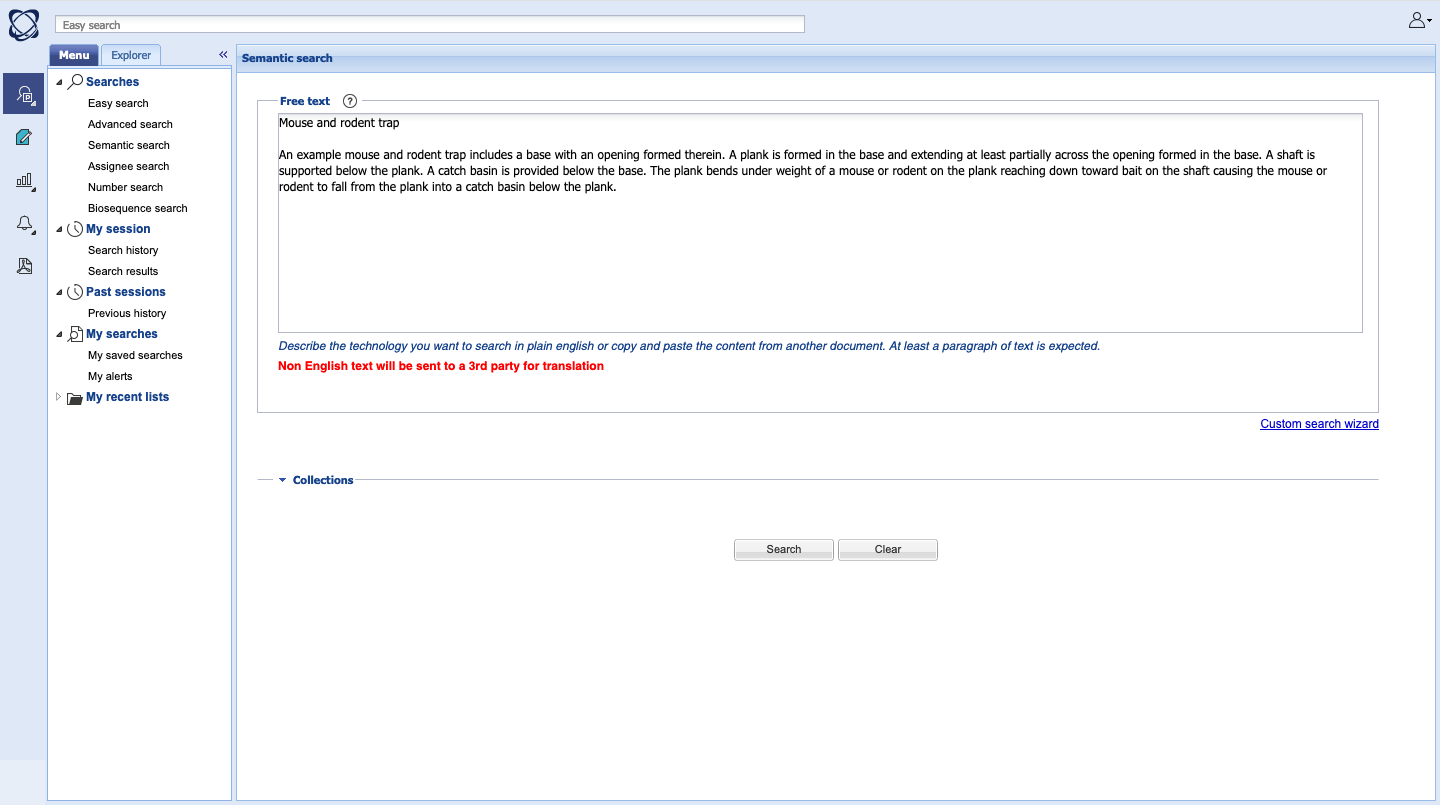The image displays a settings page of a computer application. The background is light blue with a white foreground displaying text predominantly in black. The top of the page features a menu with options such as "Explore" and "Semantic Search." Under "Searches," there are several categories including "Easy Search," "Advanced Search," and another which is slightly illegible due to the small and fuzzy text. Additional options visible on the page are "Search History," "Search Results," "Past Sessions," "My Results," "My Saved Searches," "My Data," and "My Recent Lists."

The main section of the interface showcases a detailed description of a mousetrap mechanism. It describes a base with an opening, and a plank extending across this opening. A shaft is supported below the plank, and a catch basin is positioned beneath the base. The text explains that the plank bends under the weight of a mouse or rodent attempting to reach bait on the shaft, causing the animal to fall into the catch basin.